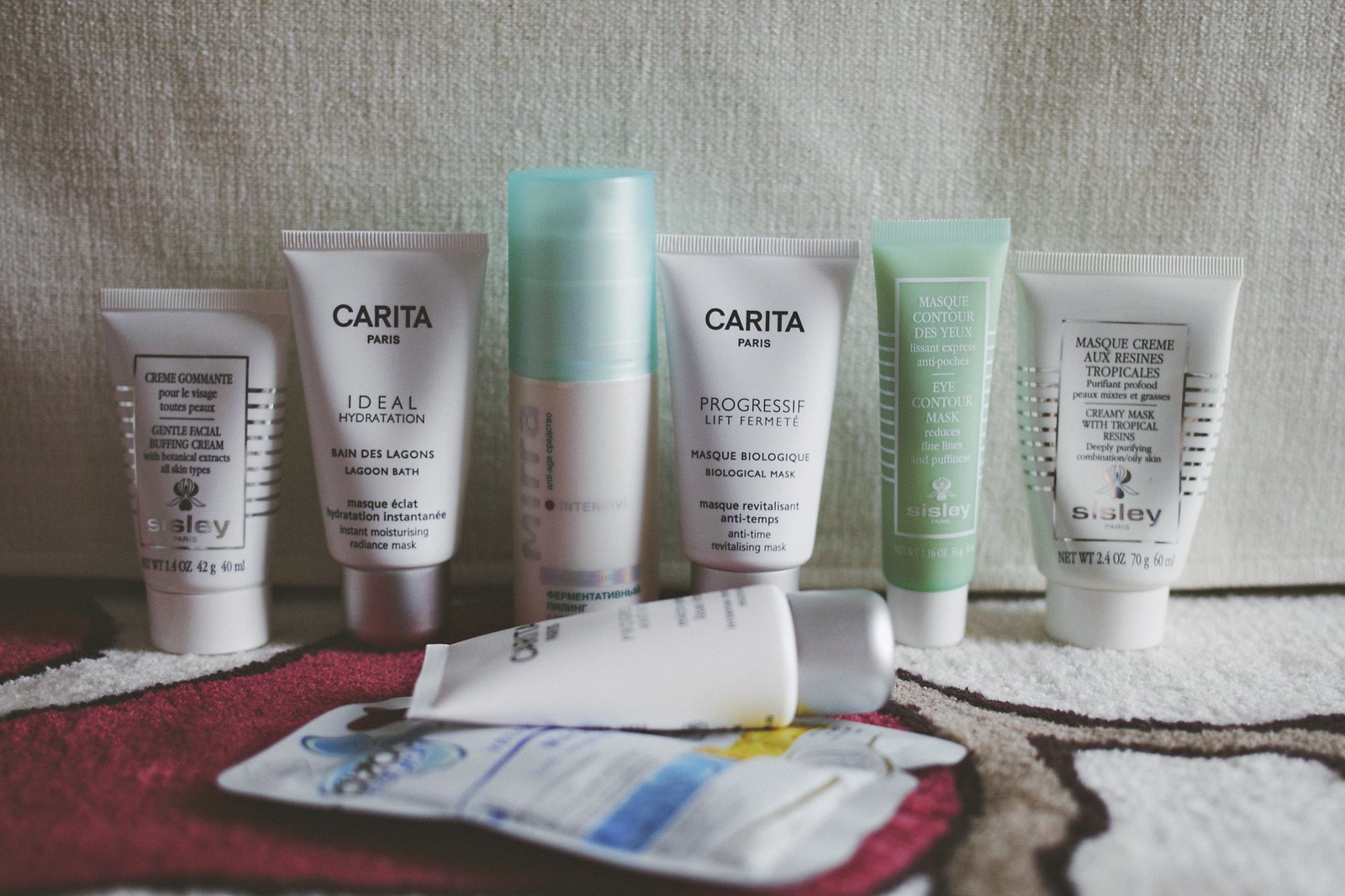The photograph captures an arrangement of various toiletries placed on a white surface with a design partially obscured by the items, featuring gray and red accents outlined in black. The visible toiletries include several packets and tubes positioned in two distinct rows.

In the foreground, a single packet with an unreadable label and a small white tube with a gray lid are prominently displayed.

Behind these, a neat row of six bottles and tubes are carefully lined up, all of which appear to be skincare products:

1. A small white tube labeled "Gentle Facial Buffing Cream" from Sisley, weighing 4 ounces.
2. Another white tube with the label "Carita Paris Ideal Hydration Lagoon Bath."
3. A white bottle with a blue lid, adorned with text that is difficult to read.
4. Another product from Carita Paris, labeled "Progressif Biological Mask."
5. A green tube with a white lid, labeled "Eye Contour Mask" from Sisley.
6. Finally, a white tube with silver stripes labeled "Creamy Mask with Tropical Resins" from Sisley, with a net weight of 2.4 ounces.

Each item is meticulously placed, highlighting the variety of luxurious skincare products.